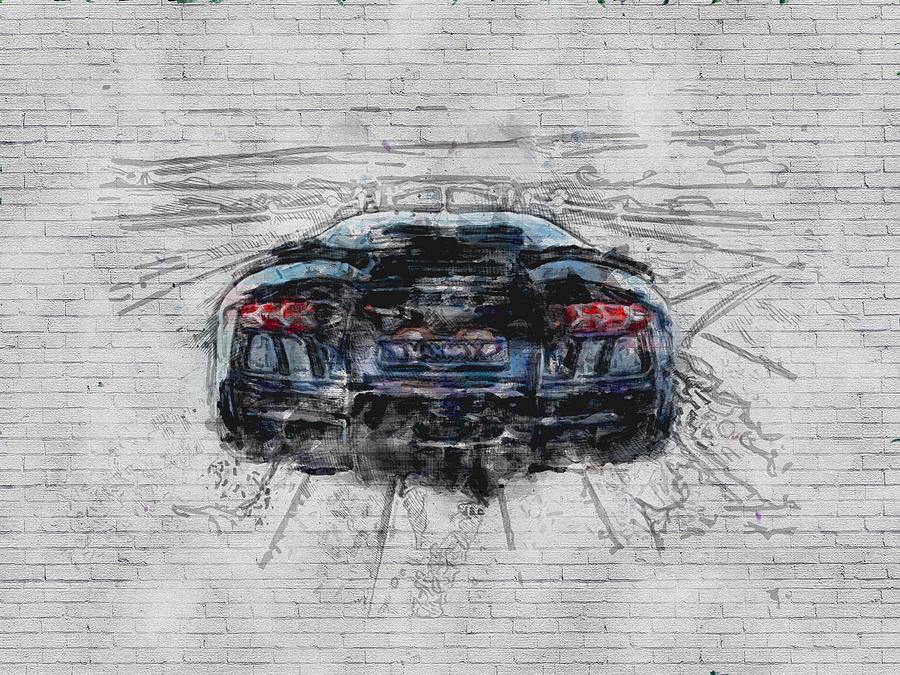The photograph captures a hand-drawn mural on a large brick wall, entirely painted in an off-white color. The centerpiece of the mural is the rear view of a high-end sports car, possibly a Ford Mustang or BMW, depicted in dark blue with vivid red taillights and a black bumper. Despite its somewhat abstract style, the car dominates the composition. Surrounding it are light grey, sketch-like lines suggesting a road and distant landscape, including the faint outline of a bridge. At the base of the mural, the initials "JAC" or "JAO" are inscribed in black, lending a personal touch to the artwork.